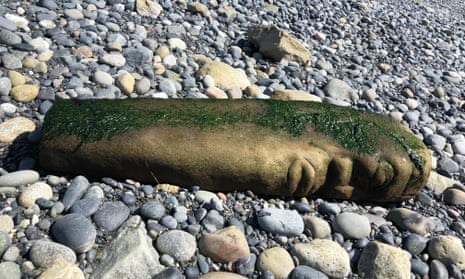In the center of this photograph, set amidst a bed of smooth, rounded pebbles typical of a lakeshore or ocean shore, lies an intriguing oblong stone with a detailed carving. The stone, possibly made of dark brown sandstone or perhaps quartz, depicts a face with discernible lips, nose, and eyes. The carving extends along the narrow, slightly pointed surface of the stone, giving it a totemic appearance that might suggest some ancient cultural or religious significance. The stone's surface is otherwise smooth, except for the distinctly carved facial features. A noticeable layer of green moss or algae covers one side of the stone, indicating it has been submerged in water recently. This environmental interaction adds depth and texture to the overall scene, accentuating the stone's worn and enigmatic presence among the gray, beige, and brown pebbles that surround it.